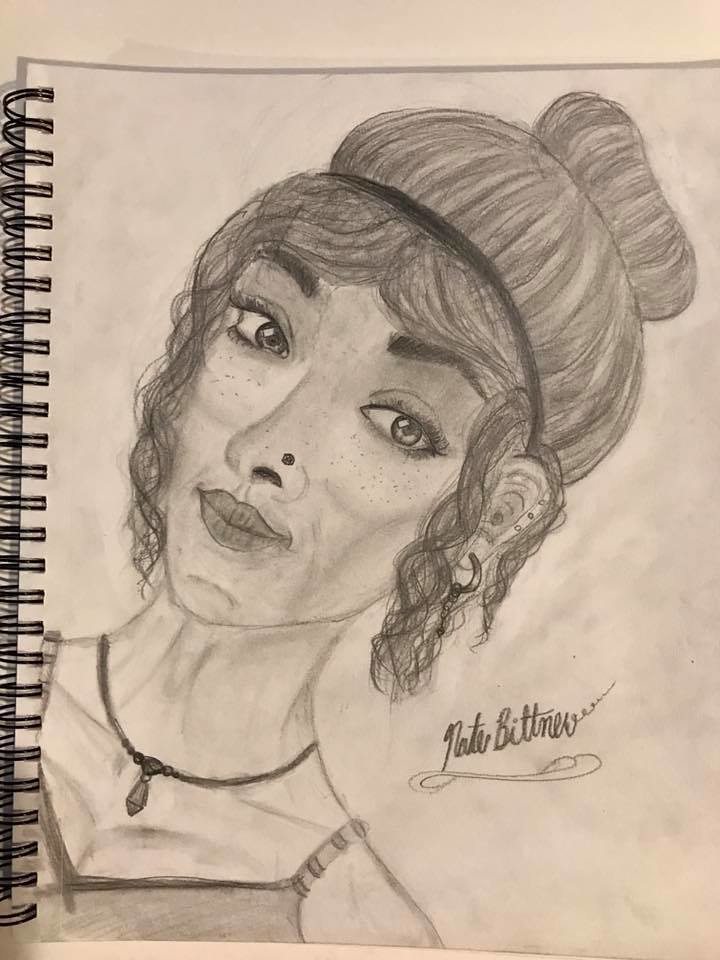This photograph captures a sketchbook with a spiral binding, open to a page featuring a highly detailed black-and-white portrait of a woman. The portrait, signed by Nate Bittner, presents the woman in a striking diagonal composition that occupies almost the entire page, from her head and face to her upper shoulders. Her hairstyle is intricately depicted, with a thin ribbon or hair band situated just above her bangs. Her long hair is styled into a bun atop her head, with curtain bangs and delicate ringlets gracefully framing her face and hanging down near her ears. A small mole can be observed on the left side of her nose, adding a touch of realism to her bright, expressive eyes. The overall impression suggests that the woman has a slender physique.